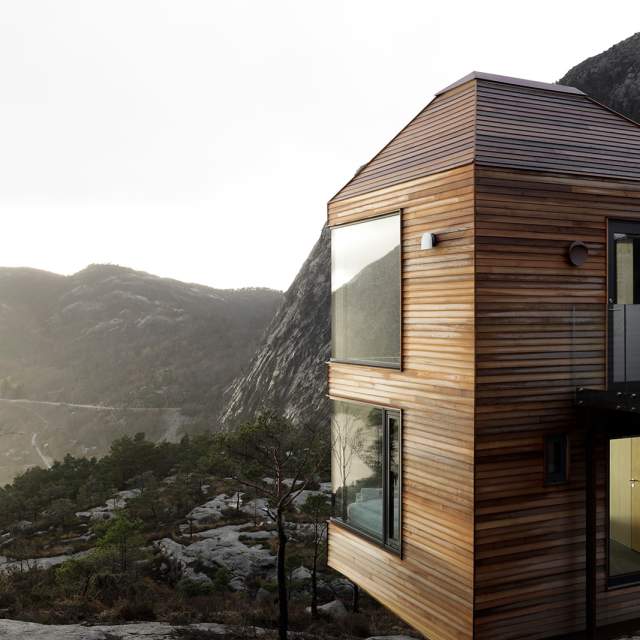In this captivating photograph taken in the heart of nature, a unique vertically-stacked house is prominently featured on the right side of the frame. The structure of the house is reminiscent of a cube, emphasized by its vertical orientation rather than a traditional horizontal spread. The building boasts horizontal white paneling complemented by brown wood accents, giving it a modern yet rustic appearance. The house, seemingly two stories tall, has an angled roof that adds a touch of architectural flair.

Windows on both floors of the house offer a glimpse into the interiors, revealing a cozy white bed in one of the rooms, and providing an intriguing view of the picturesque landscape beyond. The background is dominated by a mountainous range, where the earthy green of foliage intermingles with the stark gray of stone, creating a striking contrast. Above, an overcast gray sky looms, adding a moody atmosphere to this serene and captivating outdoor scene.